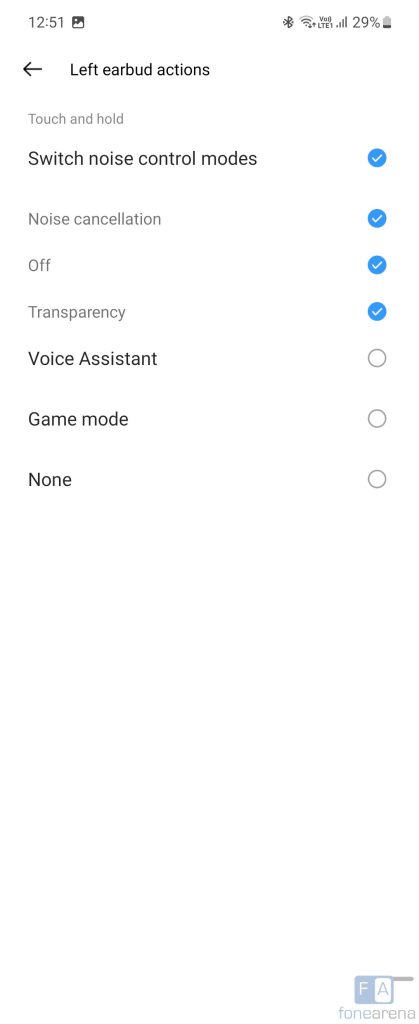This is a detailed screenshot from a cell phone displaying settings for left earbud actions. At the top left corner, it shows the time as "12:51," along with a photo icon. To the far left, there is a Bluetooth icon, signal bars, and battery life indicator showing 29% remaining. Below these icons, there is a black arrow pointing to the left.

The main section of the image lists the settings for "Left Earbud Actions" with the instructions "Touch and hold." The options under "Switch noise control modes" include:

- Noise Cancellation (checked)
- Off (checked)
- Transparency (checked)

Additionally, other options listed are:
- Voice Assistant
- Game Mode (None)

At the very bottom of the image is a logo comprising a square divided into two halves: the left half is gray with a white "F," and the right half is white with a gray "A." Beneath the logo, the text "F-O-N-E-A-R-E-N-A" is written.

The image is predominantly vertical and contains no photographic elements, people, animals, birds, or fish.